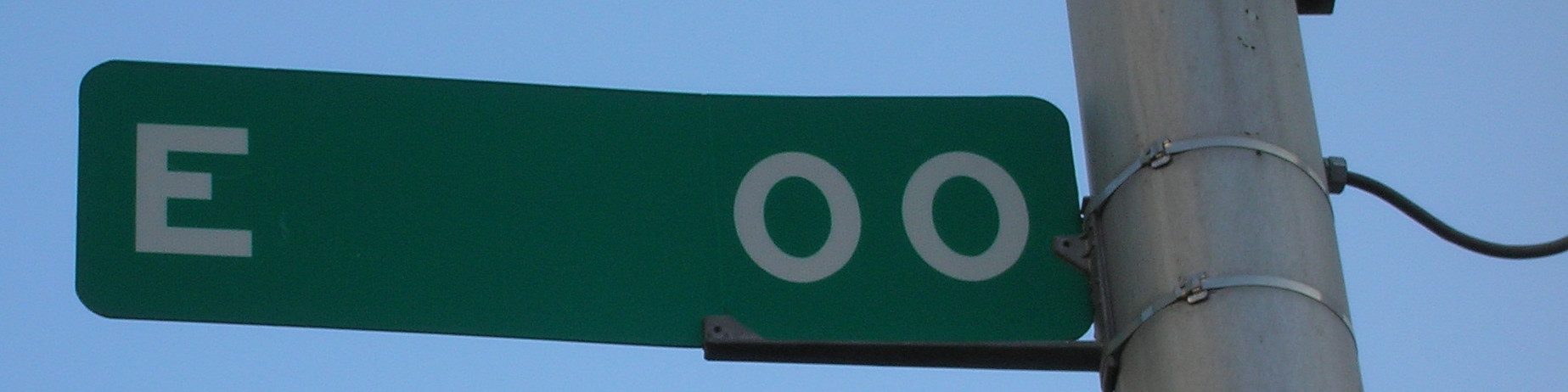This detailed photograph captures a zoomed-in view of a cylindrical, silver metal utility pole positioned on the right side of the image against a solid, cloudless light blue sky. The pole features two metallic zip ties securing a rectangular, dark green sign with rounded edges, extending to the left. A black cable is seen coming out of the pole toward the right. The sign, which appears gray in the light, displays white text: an uppercase 'E' on the far left, followed by a large blank space, and concluding with '00' near where the sign meets the utility pole.